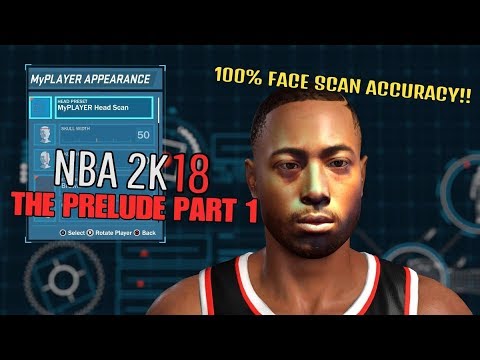This image is a still from a video game website, specifically from the interface of a computer or video game, with a focus on character customization. The background is predominantly black, providing a stark contrast to the interactive elements present. 

On the left side, there's a vertical rectangular section. It is divided into two main segments. At the top, there is a dark blue banner with the text "MyPLAYER APPEARANCE." The text is stylized with "My" in capital M and lowercase y, directly followed by "PLAYER" in full capital letters, with no space between "My" and "PLAYER." The word "APPEARANCE" is also fully capitalized.

Below this banner, there is a larger blue square divided into five different panels. The first panel contains the text "MyPLAYER HEAD SCAN." 

The second and third panels each display a human head. The second panel includes the number "50," while the third panel is partially obscured by a stamp with the text "NBA 2K18" in white print, except for "18," which is in red. Directly below this, in capitalized letters, it reads "THE PRELUDE PART 1."

In the remaining space, the graphic features a man shown from the shoulders up. He is wearing a black jersey accented with a thin orange line and a thicker white line. Above his image, the text "100% FACE SCAN ACCURACY" is displayed in yellow print, emphasizing the game's commitment to realistic character depiction.